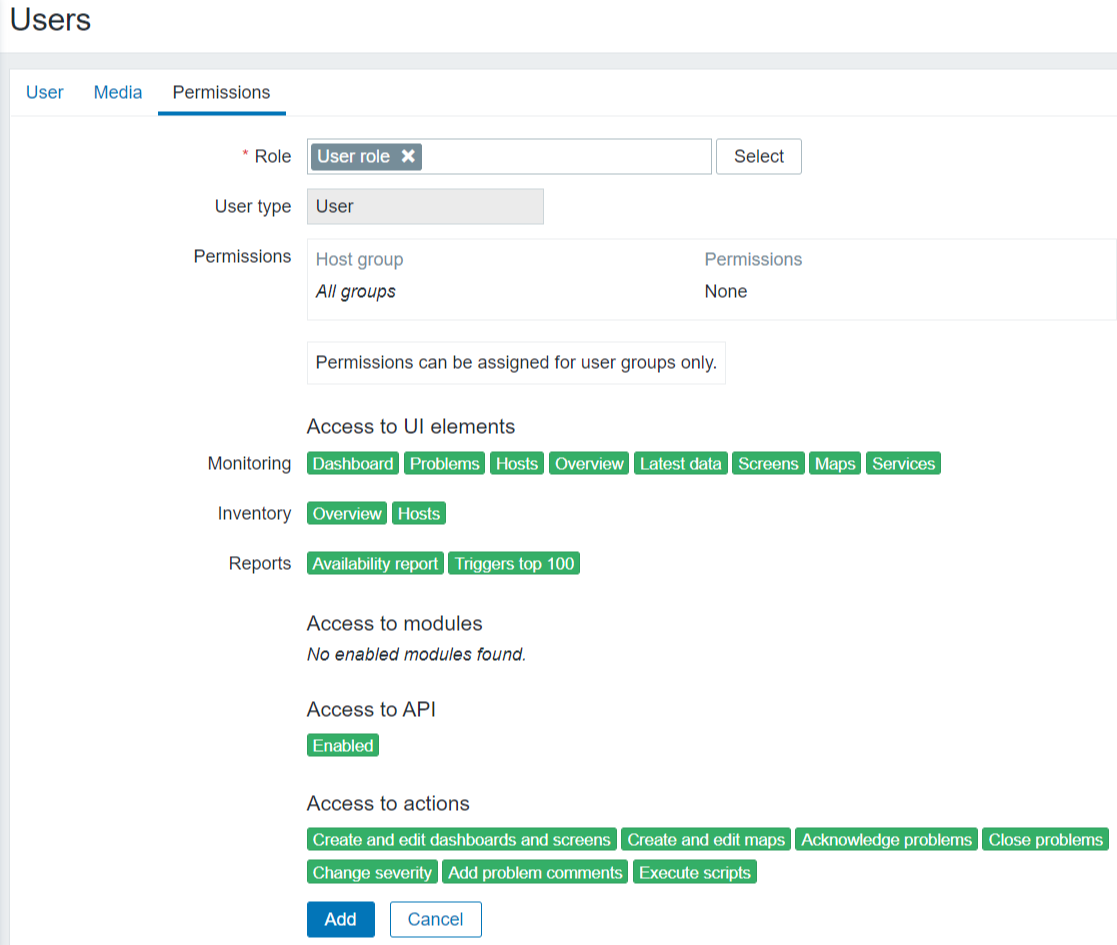Screenshot of the Administration Portal for a Website

This screenshot captures the backend of a website, displaying the administration portal designed for managing user permissions. The interface has a clean white background. The top left corner features the word "Users" in black text, indicating that the user is currently on the "Users" tab.

Below the main tab header, there are three secondary options: "User," "Media," and "Permissions." The "Permissions" option is highlighted in black text with a blue underline, signifying that the user is currently editing permissions for particular users or roles.

Central to the screen are multiple settings related to user roles and permissions. These settings include categories such as "Role," "User Type," "Permissions," "Monitoring," "Inventory," and "Reports." Each category can be edited to add or remove specific permissions tied to particular users.

The section for "Monitoring" stands out, featuring eight green boxes next to it that represent different capabilities within this role. These boxes are labeled with titles such as "Dashboard," "Problems," "Latest Data," and "Screens," indicating various functionalities that users can be granted or denied access to.

By adjusting these roles and their associated permissions, administrators can control the level of access and the range of actions that users can perform within the website's backend. This granular control ensures that users have the appropriate permissions needed for their responsibilities while maintaining the website's security and integrity.